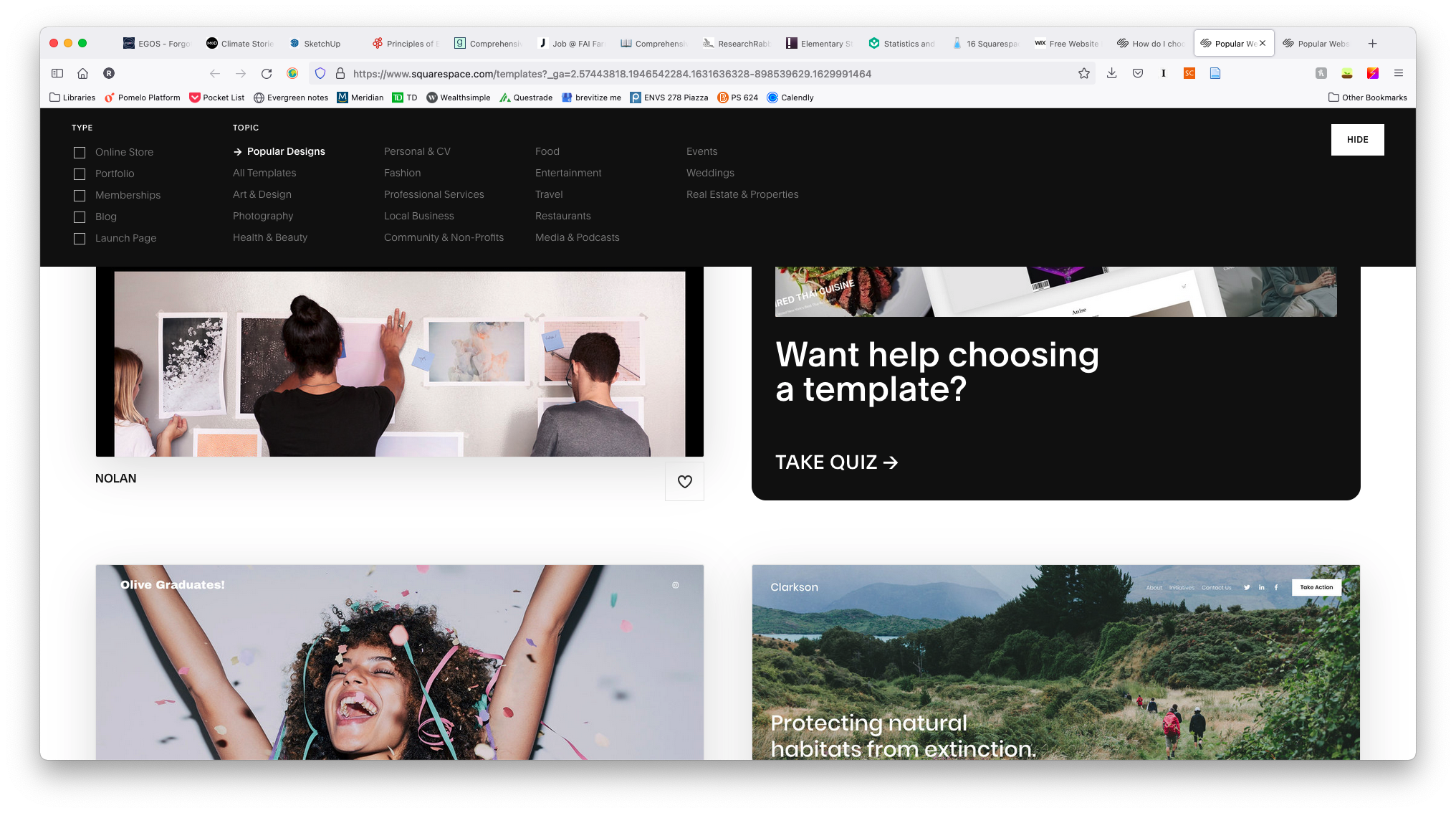The webpage features a clean white background with a central focus on four distinct images. 

In the first image on the left, three individuals—two women and one man—are engaging in an interactive activity with artworks. The central figure, a woman with her dark hair styled in a bun, wears a black t-shirt and is placing her hand on one of the art illustrations taped to the wall. To her left, another woman with brownish blonde hair in a white t-shirt appears to be removing a piece of paper from the wall. On the right-hand side, a shorter man with dark hair and a gray t-shirt is looking downwards toward the pictures, with his head angled down, intently focusing on something.

Adjacent to this, there is a prominent text box with a thick black border at the bottom. The white text within the box reads, "1. Help choosing a template. Take quiz."

Below that are two additional boxes. The box on the left features an image of a light-skinned Black woman with a curly afro, celebrating exuberantly with both arms raised. Superimposed on her image are celebratory ribbons and papers, with the text "Olive graduates. She's so happy." Her mouth is open as she screams for joy.

The adjacent box showcases a picturesque nature scene with lush mountains and expansive greenery under a clear blue sky. The top left corner of the image is labeled "Clarkson," while the bottom left corner carries the text, "Protecting natural habitats from extinction." Four individuals can be seen hiking amidst this serene landscape.

The webpage, likely linked to template designing, as suggested by the URL "HTTPS www.squarespace.com/templates" displayed in the search bar, does not overtly specify its purpose but implies a connection to creative and nature-oriented content.